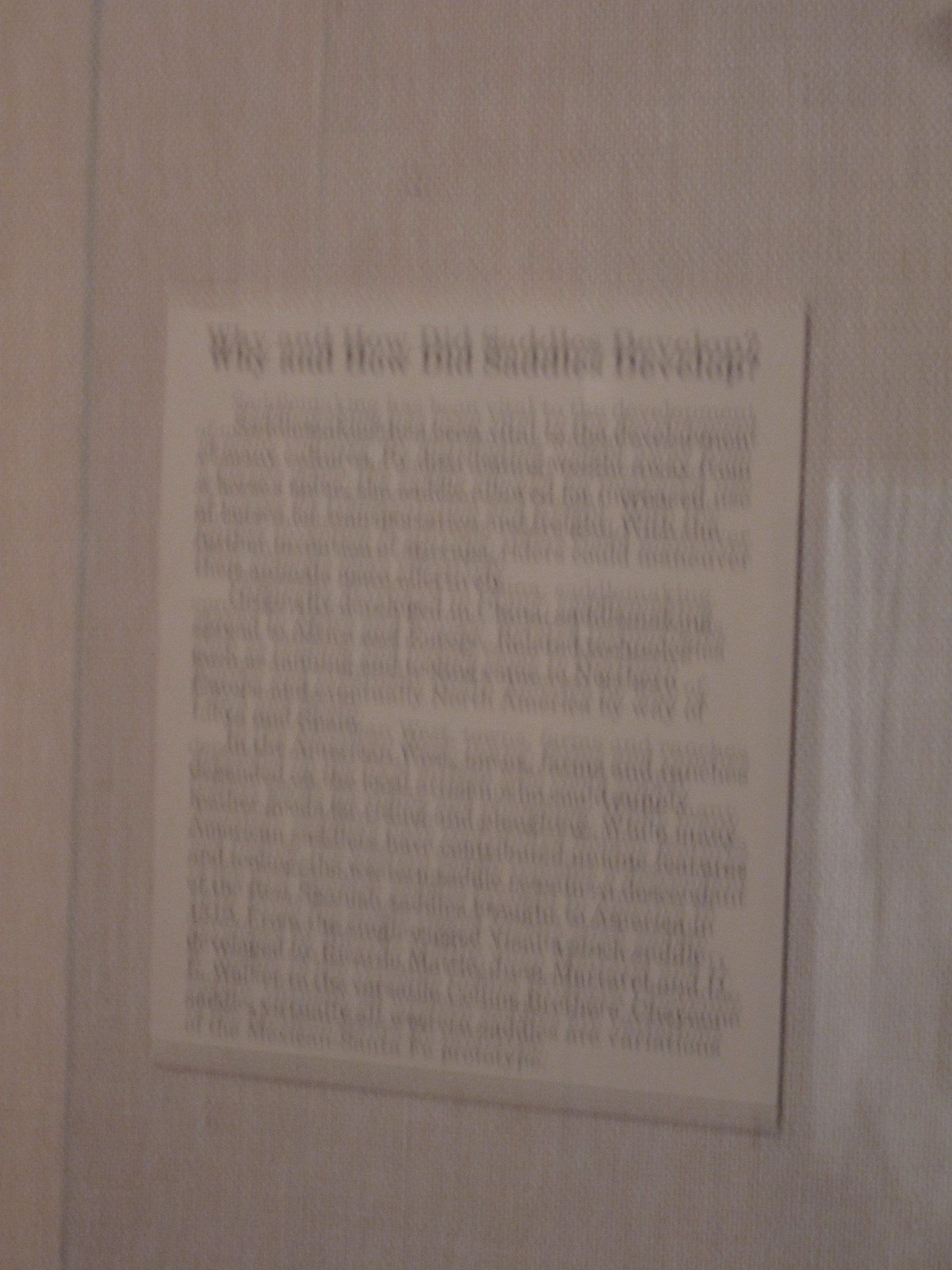The image captures a sign mounted on a paneled wall, likely the exterior of a building. Due to the camera shaking or movement, the photograph is blurry, making the text nearly illegible. However, some larger letters at the top of the sign can be discerned, reading, "Why and How Did Saddles Develop?" This suggests the sign pertains to the historical development of saddles, and it implies that the location might be a museum or exhibit focused on Western themes, possibly involving horses or saddles. The background color of the image is a light tan.